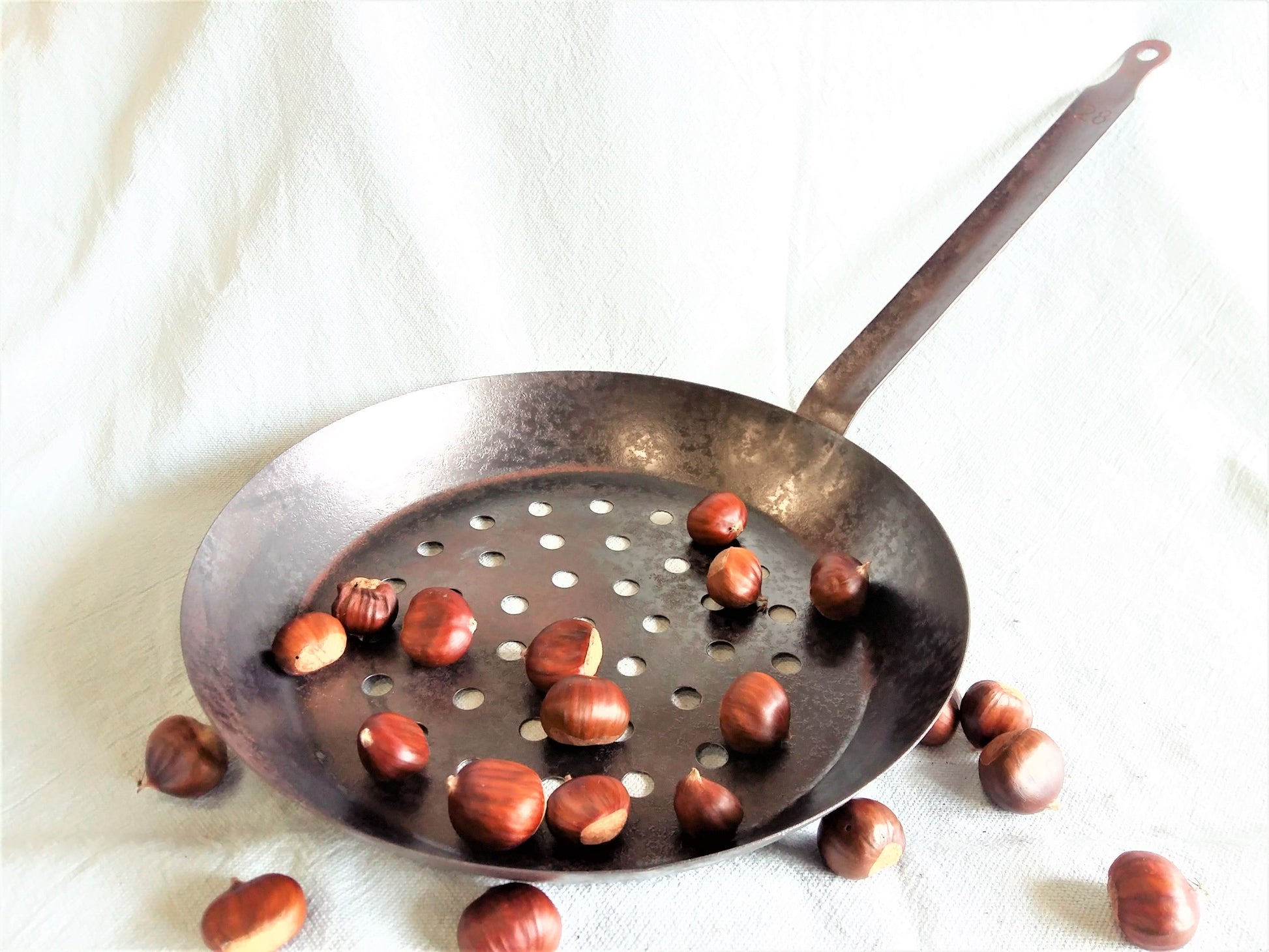The photograph depicts a well-lit scene of an iron skillet, with both the iron skillet itself and numerous chestnuts being the primary subjects. The skillet, which is circular and shallow with a long handle featuring a small hole at its end, sits on a white tablecloth. The iron skillet has a black and gray appearance with some signs of rust and use, but it is not excessively dirty or worn out. Perforations, or small circular holes, are visible on the bottom of the skillet, and it is casting a slight shadow to the left, indicative of a sunlit setting. Inside the skillet are around 10 to 15 chestnuts, their reddish-brown shells glinting in the daylight. Scattered outside the skillet on the white tablecloth are an additional 7 or 8 chestnuts, contributing to the overall rustic and cozy atmosphere of the image. The handle of the skillet bears the number "28" engraved on its surface.